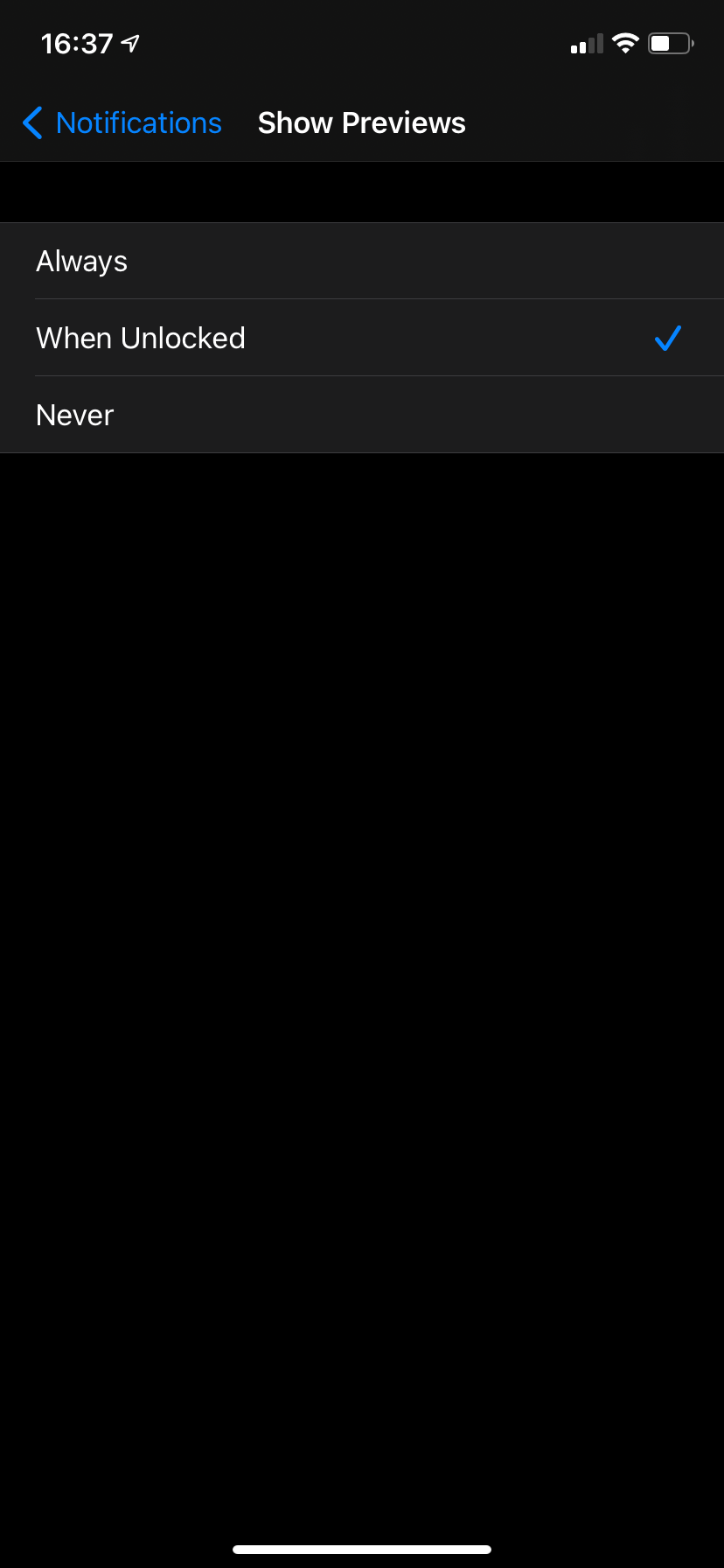The screenshot displays an iPhone with dark theme enabled, currently in the process of configuring notification settings. The background is predominantly dark grey with light grey and blue text elements. At the top of the screen, the status bar reveals the military time "16:37" on the left, alongside an active location symbol. On the right, there are indicators for mobile data strength (two out of four bars), WiFi connectivity (three bars), and battery life (at 50%).

The settings interface shows "Notifications" in blue text with an interactive blue arrow pointing left. Below this, "Show Previews" is written in white text, followed by three selectable options: "Always," "When Unlocked," and "Never." The current selection is marked by a blue check mark next to "When Unlocked."

The rest of the screenshot is mainly dark grey space, with the exception of the iPhone’s bottom navigation bar, which is white and indicates the option to pull up the recent menu or switch to other open apps. The overall layout is simple and uncluttered, focusing on the configuration options.